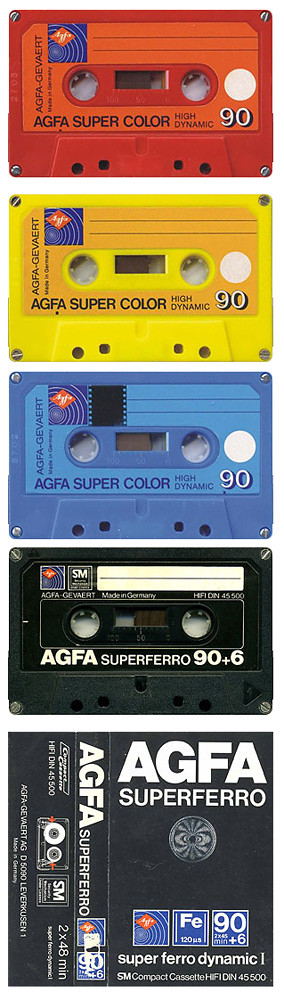The image displays a vertical stack of four vintage cassette tapes, reminiscent of the 1970s or 1980s. From top to bottom, the cassettes are colored red, yellow, blue, and black. The first three cassettes, labeled "AGFA Supercolor," are high-density, 90-minute tapes in red, yellow, and blue respectively, and also feature the "AGFA Granite" branding. The black cassette at the bottom is labeled "AGFA Superfaro 90 plus 6." Beneath the stack, a square logo advertises "AGFA Superfaro Dynamic," accompanied by additional details including "two times 48 minutes" and blue boxes with red diamond shapes. The unique design and branding details, such as "FE" and the number "90," suggest an advertisement or clip art style image, emphasizing the retro aesthetic of the cassette collection.